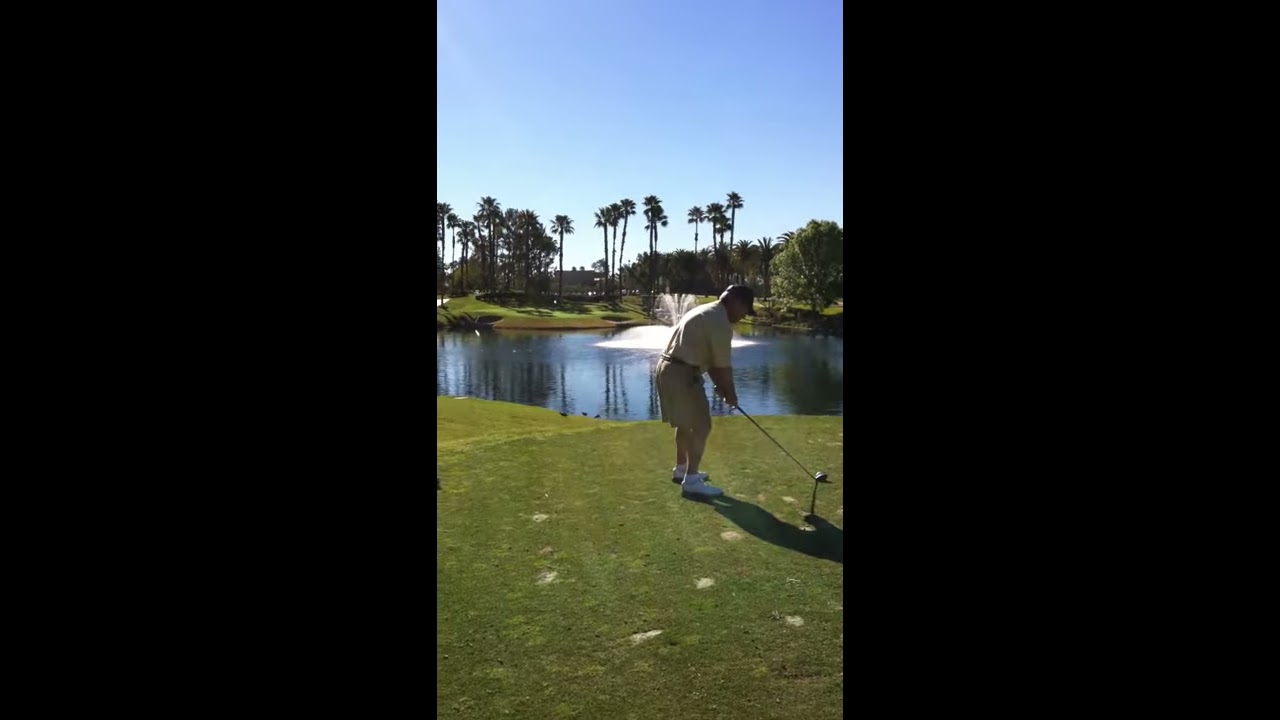A digital photograph captures an older gentleman poised to tee off on a bright, sunny day with a clear blue sky. Seen from behind, he is slightly hunched over, focusing intently on the golf ball. He wears a light tan, short-sleeved shirt, beige shorts, white sneakers, and a cap. The vivid green grass around him contrasts with a large water trap directly ahead, featuring a central fountain spewing water. In the backdrop, towering palm trees stretch skyward, flanked by shorter, lush green trees to the right. The scene is serene and picturesque, underscored by the solitary golfer preparing his drive over the expansive pond.